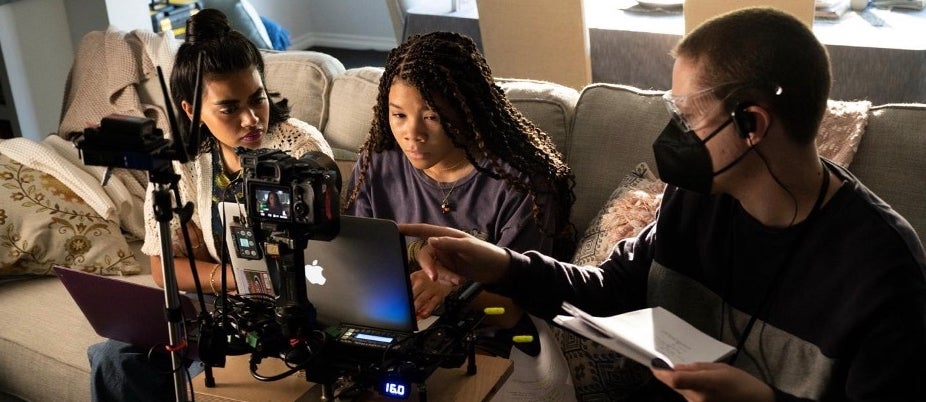The photograph, taken indoors during the daytime, captures a scene with three people sitting on a light tan tweed couch, adorned with blankets, pillows, and draped sweaters. The couch faces a table, upon which rests an Apple laptop and a couple of cameras. The central figure is a young girl of African descent with long, wavy black hair styled in thin braids. She wears a purple shirt and is intently focused on the laptop in front of her. To her left sits another girl, likely of Indian descent, with brown skin, dark hair pulled into a bun on top of her head, and the rest cascading around her shoulders.

On the right of the photograph is a young Caucasian man with short, cropped, light-colored hair. He wears clear safety glasses, a black face mask, and a black earpiece. In his left hand, he holds some papers while his right hand points towards the laptop, indicating he is guiding or instructing the two girls. The equipment setup, including multiple cameras pointed at the girls, suggests the group is engaged in an activity like podcasting or video recording.